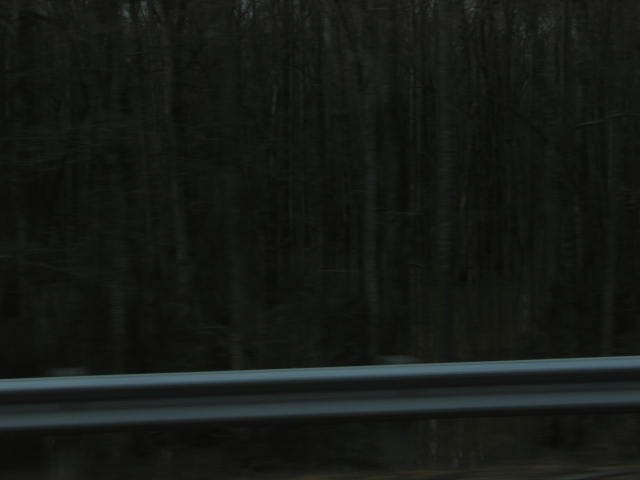The image largely obscured by darkness captures a blurry nighttime scene of a dense forest. Slender, grayish-white trees with hanging moss dominate the landscape, standing side by side with little light penetrating their dense formation. In the foreground, a highway guardrail runs horizontally across the frame, with two vertical beams supporting it. The scene behind this metal barrier fades into inky blackness, further emphasizing the mysterious depth of the forest. The guardrail, a clear indicator of a roadside view, juxtaposes the structured human element against the untamed natural setting.